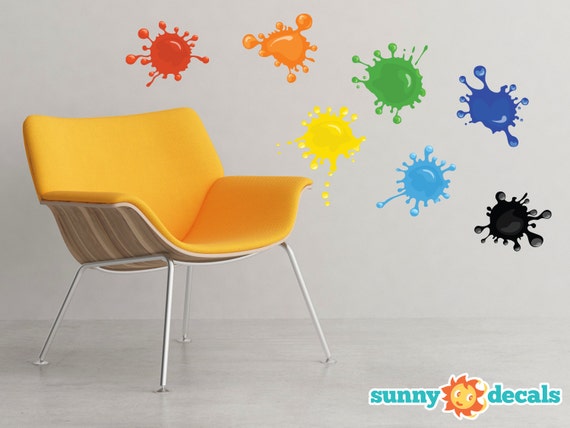This advertisement for Sunny Decals features a single, low-seated chair, possibly designed for children, with a light orange cushion and backrest. The chair stands on thin, silver-colored metal legs with a light brown underside accented by darker brown stripes. The smooth, shiny floor beneath it is gray, matching the light gray, solid-colored wall in the background. Prominently displayed on this wall are seven digitally rendered paint splatters in the colors red, orange, yellow, green, light blue, dark blue, and black, resembling the whimsical shapes of germs. In the bottom right corner of the image, the “Sunny Decals” branding is shown in small aqua letters, accompanied by a cheerful sun icon with a smiley face and radiant flames.